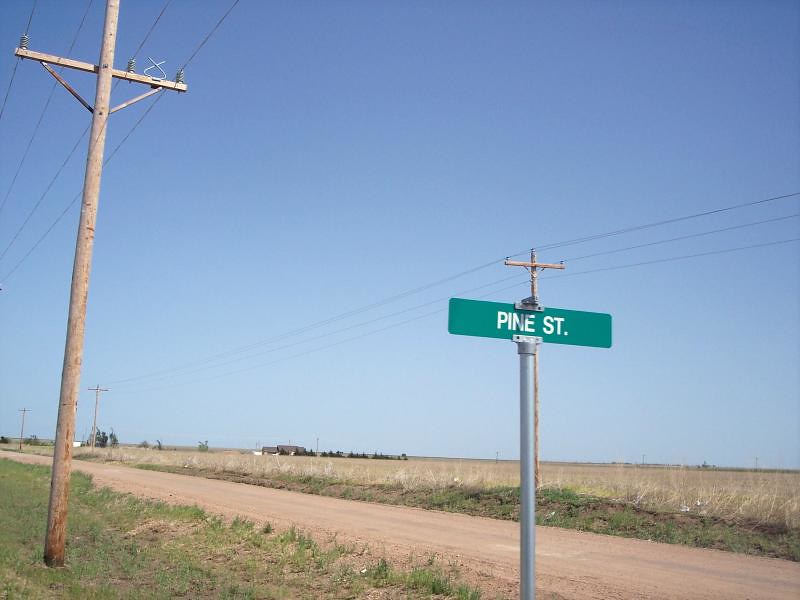A rural dirt road extends horizontally across the scene, intersected by tall power poles and phone lines on either side. Prominently visible is a green street sign reading "Pine Street" in white text, mounted on a vertical silver metal post and located in the right half of the image, around the midpoint. The road starts from the lower right corner and progresses slightly higher toward the left due to perspective. Overgrown grass in a shallow ditch occupies the foreground, contrasting with the elevated grassy dirt on the other side of the road. Beyond this, a flat, expansive field filled with tan crops, likely wheat, stretches into the horizon. Left and right power line posts flank the road, each supporting four parallel electrical wires. In the distance, the horizon is dotted with a few trees and a lone house, accentuating the vast, open landscape devoid of hills or mountains.